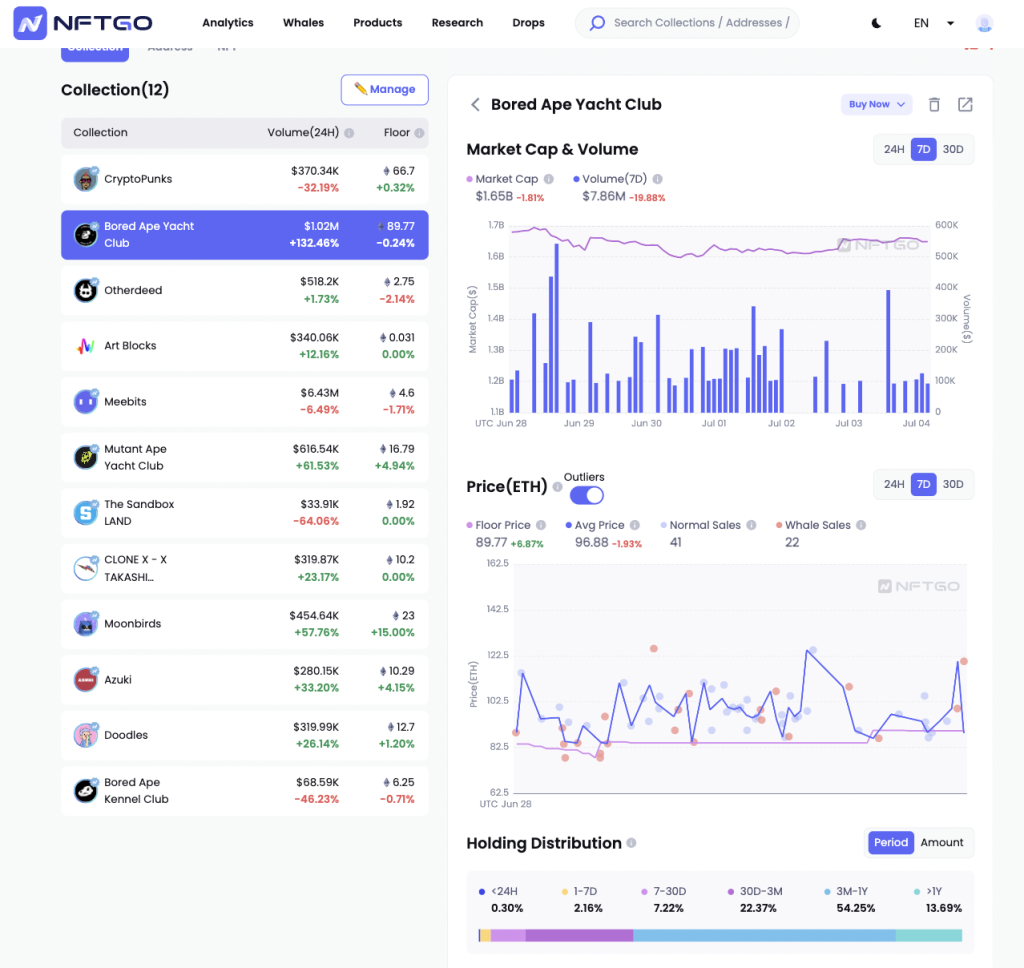The screenshot captures a comprehensive dashboard of an NFT (Non-Fungible Token) analytics platform named NFT Go. In the top left corner, there's a stylized logo featuring a purplish blue square with a prominent white letter "N." Next to the logo, the text "NFT Go" is displayed, accompanied by a row of navigational links labeled: Analytics, Whales, Products, Research, and Drops. Further right, a search bar is visible beside a crescent moon icon, indicating a possible dark mode toggle. Beyond these, there’s a language selection drop-down menu and a circular user profile icon.

Beneath the navigation bar, the section is titled "Collection," with the number "12" in parentheses, hinting at the number of items in the user's collection. Adjacent to this is a "Manage" button. Below, various columns are presented, listing users, volumes, and their respective positive or negative percentage changes. 

On the right side of the screenshot, the "Bored Ape Yacht Club" collection is featured with actionable buttons: "Buy Now," "Trash," and "Forward." Market cap and volume metrics are displayed, with options to view data over 24 hours, 7 days, or 30 days. A detailed graph illustrates the performance of the stock/collection.

Further down, there is a section titled "Price (ETH)" highlighting outliers, showcasing metrics such as floor price, average price, normal sales, and wholesales. This section includes another interactive graph populated with various data points that can be highlighted for more detailed analysis.